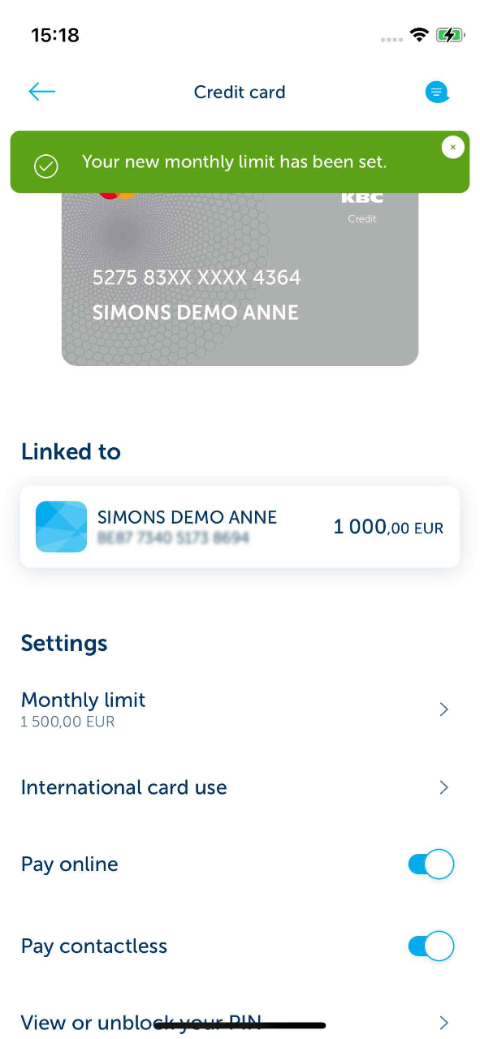Screenshot of a mobile application interface managing a credit card:

The top section of the screen displays the iPhone’s status bar. The time is 15:18 on the top left, with cellular service bars next to it, although no service is available, indicated by the greyed-out bars. The Wi-Fi signal is strong, showing 3 bars, and the battery icon is fully charged while also displaying the charging symbol.

The main interface starts with a blue back arrow on the top left, a centered title "Credit Card," and a blue chat icon on the top right. Below this header, a green banner with a check mark announces, "Your new monthly limit has been set."

The main content area features an image of a gray MasterCard with partial card number "5275 83XX XXXX 4364". The cardholder name displayed is "Simon's Demo Inn."

Following the card image, there is a section titled "Link to" which highlights "Simon's Demo Inn" in a blue box accompanied by the amount "1,000 EUR".

The settings section lists multiple options:
1. **Monthly Limit** - Displays "1,500 EUR" and includes an arrow for further actions.
2. **International Card Use** - Has an arrow indicating more settings.
3. **Pay Online** - Indicates this option is active with a toggled-on switch.
4. **Pay Contactless** - This option is also active with a toggled-on switch.
5. **View or Unblock your PIN** - Includes an arrow for navigation to additional options.